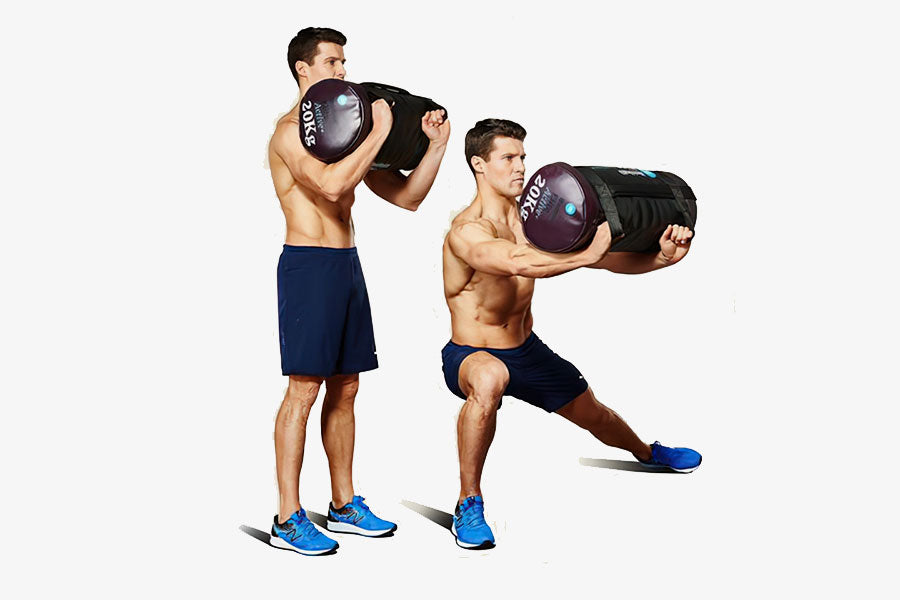The image showcases a muscular, shirtless Caucasian man with short hair, demonstrating an exercise involving a 20 kg duffel bag-like weight. The scene features two positions of the same man side by side: in the first, he stands upright, holding the bag with both arms curled under, lifting it towards his chin as if performing a bicep curl. In the second position, he adopts a dynamic pose, squatting with one leg extended to the side and the other knee bent, while holding the bag extended in front of him, emphasizing his defined arm, chest, and leg muscles. The man wears navy blue shorts and light blue sneakers, possibly New Balances, and the overall impression suggests an advertisement for this multifunctional exercise tool.